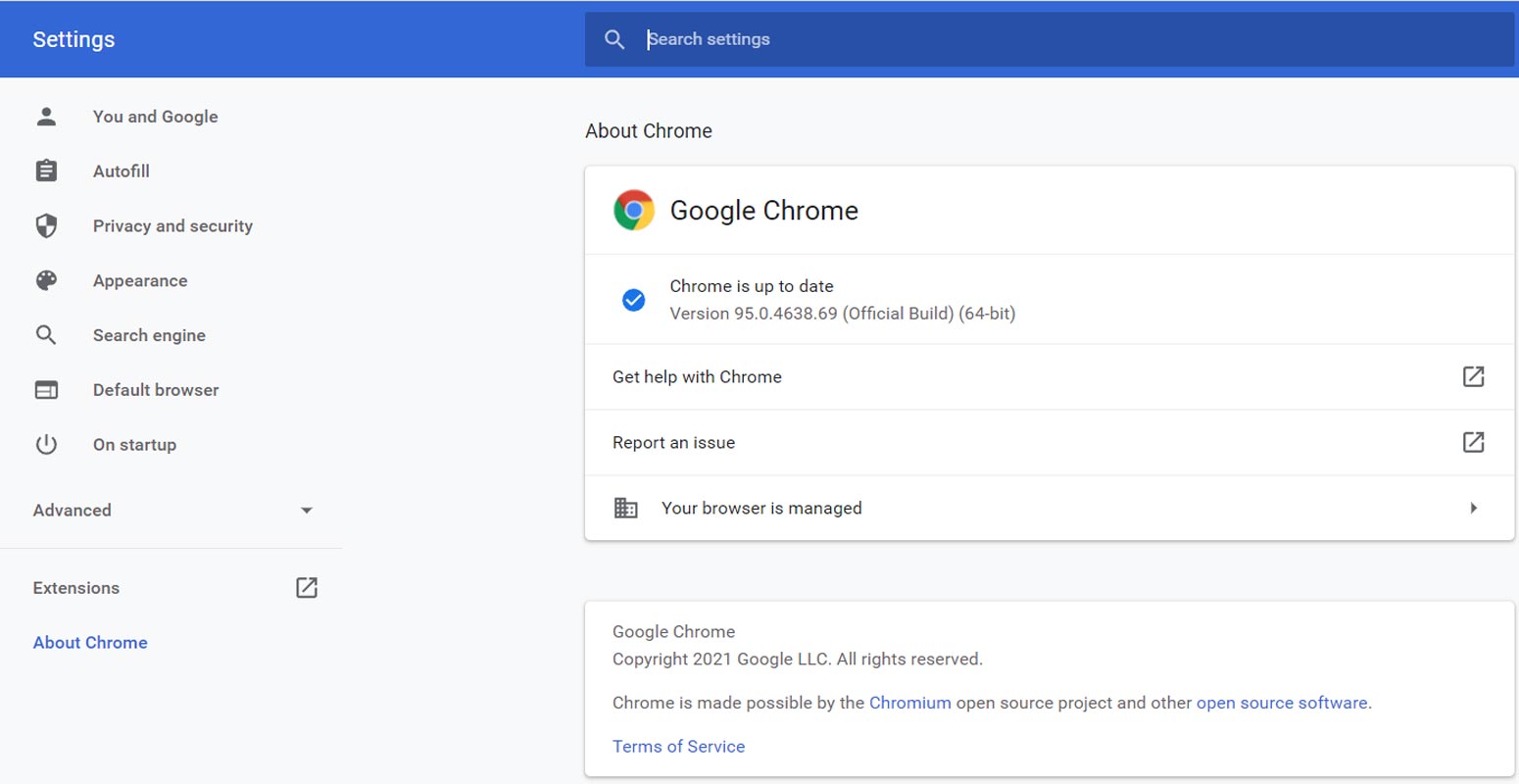The image depicts a screenshot of a webpage showing the settings menu of the Google Chrome browser. At the top part of the screen, inside a blue rectangle, the word "Settings" is prominently displayed. Next to it, near the center, is the "Search settings" bar with a visible cursor, suggesting that a user can type a query.

Down the left side of the page, there is a vertical row of icons and options. These include:
- A silhouette of a human labeled "You and Google"
- A clipboard icon labeled "Autofill"
- A shield icon labeled "Privacy and security"
- An artist's paint palette labeled "Appearance"
- A magnifying glass labeled "Search engine"
- A rectangle with lines labeled "Default browser"
- A power button labeled "On startup"

Below these options, there is an expandable drop-down labeled "Advanced." Further down, there's an "Extensions" category marked with a square and an arrow icon. Additionally, there is an "About Chrome" option, presented as a clickable blue link.

In the main area of the page, the user has selected the "About Chrome" section. Consequently, the central part of the screen displays details about Google Chrome. This includes the Chrome icon and the text "Google Chrome" followed by a check mark indicating that "Chrome is up to date." The version number of Chrome is also displayed, along with options to "Get help with Chrome" and "Report an issue."